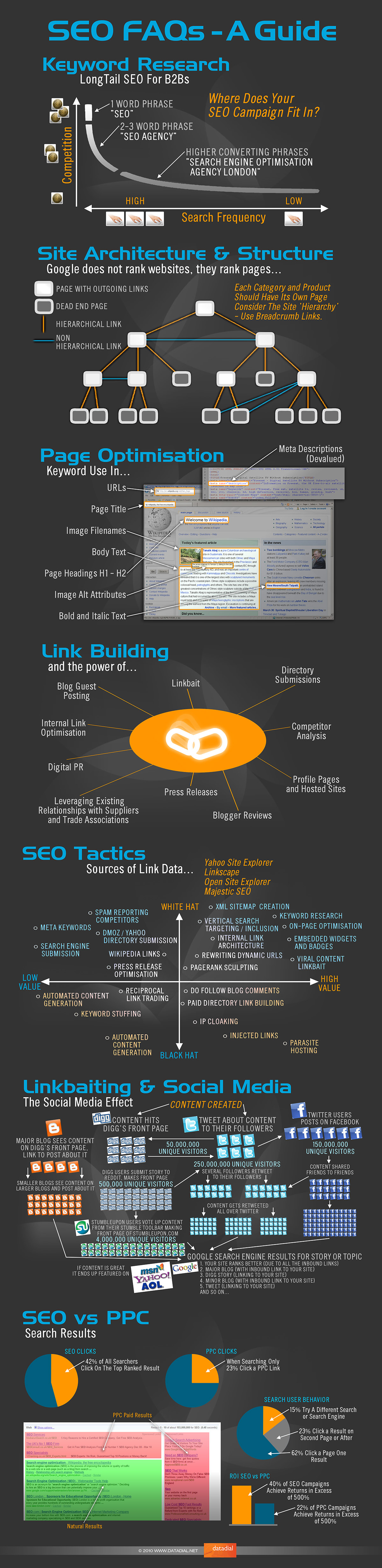This image illustrates an informative and comprehensive "SEO Frequently Asked Questions Guide," seemingly formatted as a downloadable PDF. The guide is structured as a single long page, integrating various text colors for emphasis.

At the top of the page, headers marked in blue denote each section of the guide, providing a clear structure. Detailed explanations in white text follow these headers, and key terms are highlighted in orange for emphasis.

The main sections of the guide include:

1. **Keyword Research**: This part outlines the core components of keyword research, complemented by charts and arrows demonstrating the workflow. Subsections include "Volunteer SEO" and the integration of SEO campaigns. It also discusses specific phrases and how to convert them, exemplifying terms like "SEO agency."

2. **Site Architecture and Structure**: This section presents a flowchart resembling a family tree, explaining the hierarchical organization of a website's structure.

3. **Page Optimization**: Key elements of page optimization are detailed here, with examples pointing to specific components such as URLs, page titles, image file names, and body text.

4. **Link Building**: Represented by a central pie chart, this section illustrates various link building strategies. Elements like link bait, press releases, digital PR, guest posts, and direct submissions are connected to the central concept.

5. **SEO Tactics**: A comparative analysis of high-value and low-value SEO tactics is illustrated through a left and right-sided layout. Examples of low-value tactics include meta keywords and keyword stuffing, while high-value tactics feature injected links and on-page optimization.

6. **Link Baiting and Social Media**: This section explores the relationship between content and social media engagement. Charts illustrate the process from content creation to major blog hits and subsequent social media interactions.

7. **SEO vs. PPC**: The final section uses pie charts and colored graphs (pink and green) to compare and contrast SEO (Search Engine Optimization) and PPC (Pay-Per-Click) strategies.

Overall, the guide is a visually rich and detailed resource, providing step-by-step insights into various aspects of SEO, enhanced by a mix of textual explanations and graphical aids.